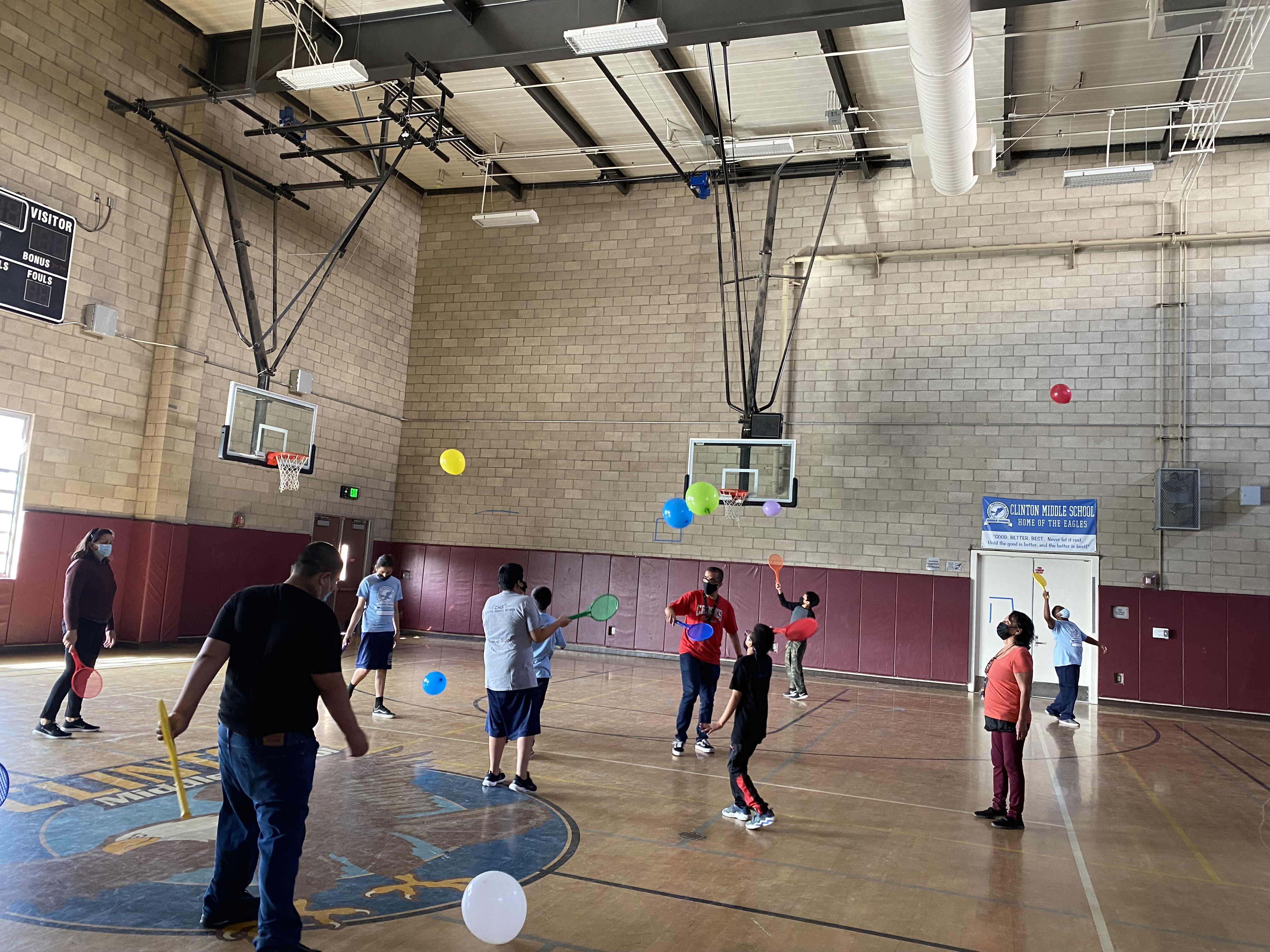The photo captures a lively scene inside a middle school gymnasium, specifically Clinton Middle School, home of the Eagles. The wooden basketball court features a large eagle mascot emblem at its center. Around ten people, a mix of children and adults, are scattered across the court, all wearing COVID masks and actively participating in a game. They hold colorful toy rackets in their hands—red, green, blue, orange, and yellow—used to swat at equally colorful balloons floating above them. The balloons are white, blue, yellow, green, purple, and red. Two basketball hoops are visible, one positioned in the upper left corner of the frame and the other toward the middle right, hanging from the high ceiling. The gym's walls are lined with maroonish-red patterned padding, above which are concrete blocks forming the structural framework. The vibrant activity and varied colors of the rackets and balloons create a dynamic and engaging atmosphere within the bustling gym.